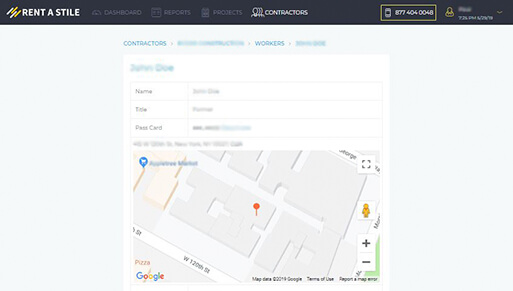This is an image of a website homepage titled "Rent a Stile," with "Stile" spelled as S-T-I-L-E. The top section of the website features a black rectangular navigation bar with clickable options labeled "Dashboard," "Reports," "Projects," and "Contractors." To the right of these options is a yellow-highlighted rectangle containing a phone number for easy visibility. Additionally, there are several blurred-out sections on the top right side of the navigation bar, likely for privacy reasons.

The primary background of the website is a light gray shade. Centrally located on the page is a prominent white box. At the top of this white box, the word "Contractors" is visible, followed by a series of blurred-out areas. Below this, the sections labeled "Workers" and "Name" are also blurred, presumably to obscure specific details. The name "John Doe" appears in one instance but is similarly blurred out in subsequent mentions, along with fields labeled "Title" and "Pass Card."

At the bottom of the white box, an unblurred map is visible, providing a means of location context within the website. This screenshot appears to be a part of an interface designed for managing various elements related to contractors and workers, with privacy considerations taken into account by blurring sensitive information.